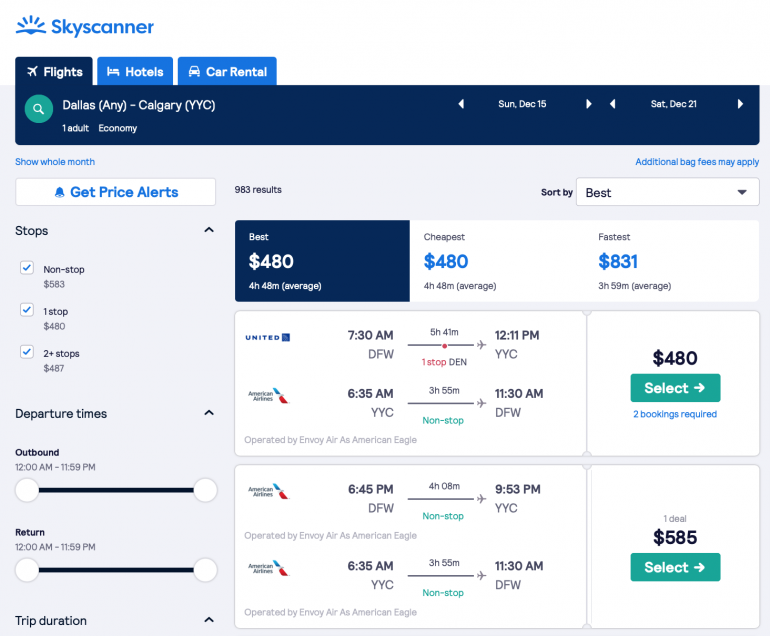This is a detailed screen capture of the Skyscanner website's flight search results page. At the top, there are tabs for various travel services, including flights, hotels, and car rentals, with the current page focused on flights. Directly below the flights tab, there is a search bar displaying the selected route, "Dallas to Calgary," along with the travel dates, "Sunday December 15th to Saturday December 21st."

On the left-hand side, a vertical sidebar offers multiple filter options, including departure and return times, number of stops (non-stop, one stop, two stops), and trip duration, each with corresponding checkboxes for selection.

The central and right sections dominate the screen with a list of flight options segmented by categories: Best, Cheapest, and Fastest. For this search:

- The "Best" flight is priced at $480.
- The "Cheapest" flight is also listed at $480.
- The "Fastest" flight costs $831.

Multiple airlines provide flight options, clearly listed with routes and return details. For example:

- One option features a departure with United Airlines from Dallas to Calgary and a return flight with American Airlines.
- Another selection shows both departure and return flights operated by American Airlines.

Each flight option includes selection buttons, allowing users to choose their preferred itinerary.